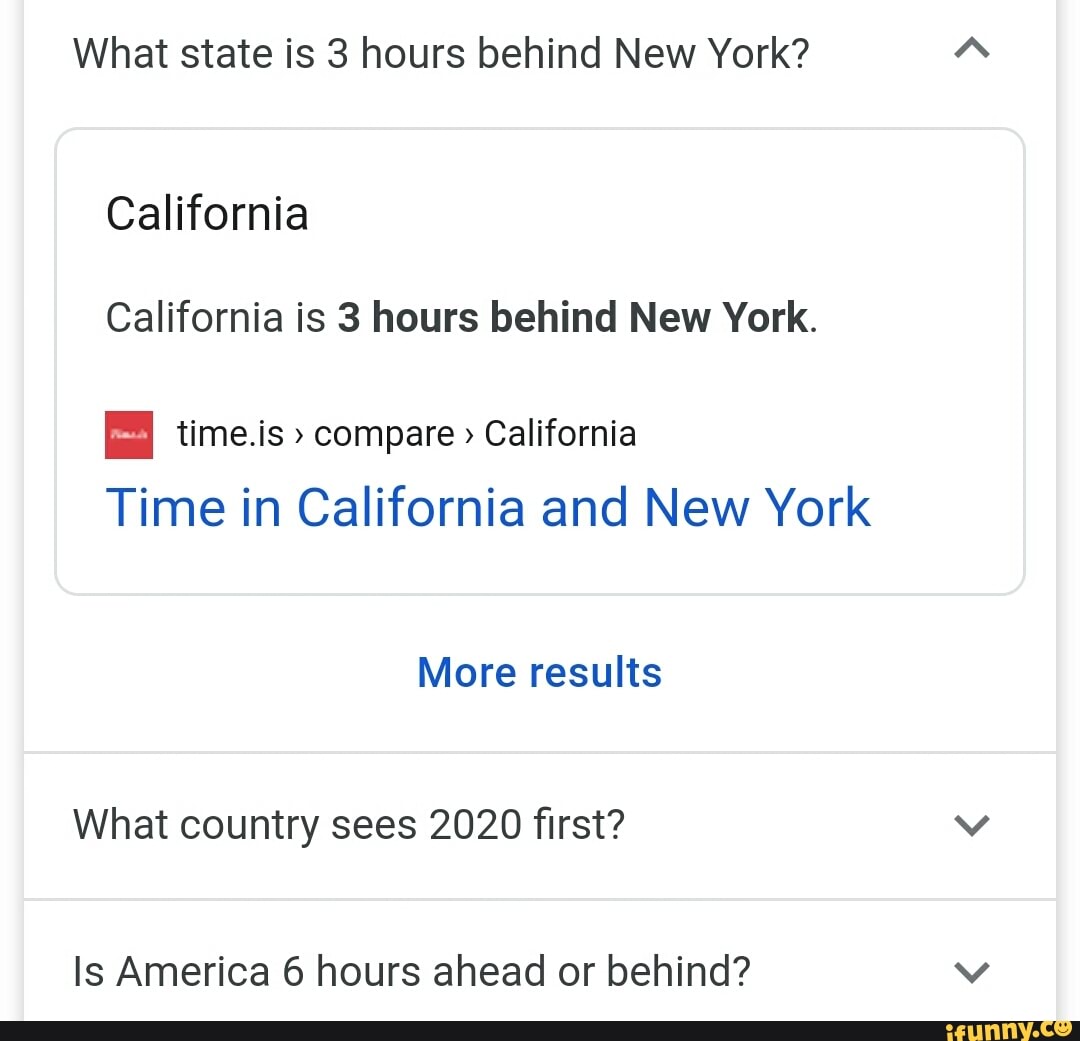This image is a cropped screenshot from a mobile device, displaying a Google search result. A black border lines the bottom of the screenshot, accompanied by a yellow watermark text from the website "ifunny.co," indicating its source. The image captures a portion of a Google search with a clean, light-colored background.

At the top of the screenshot is the search query: "What state is three hours behind New York?" The answer is provided in a small gray box that states, "California." While California is indeed three hours behind New York, the search result further includes a link to the originating website, "time.is," with a clickable blue text link reading "time in California, New York."

Below the initial result, there is an option in blue text labeled "More results," followed by two additional questions. These questions are: "What country sees 2021st?" and "Is America six hours ahead or behind?" Each question includes a drop-down arrow, suggesting that more information can be revealed by interacting with them.

Overall, the image succinctly encapsulates a specific search query about time zones, illustrating the digital interface of a mobile Google search.